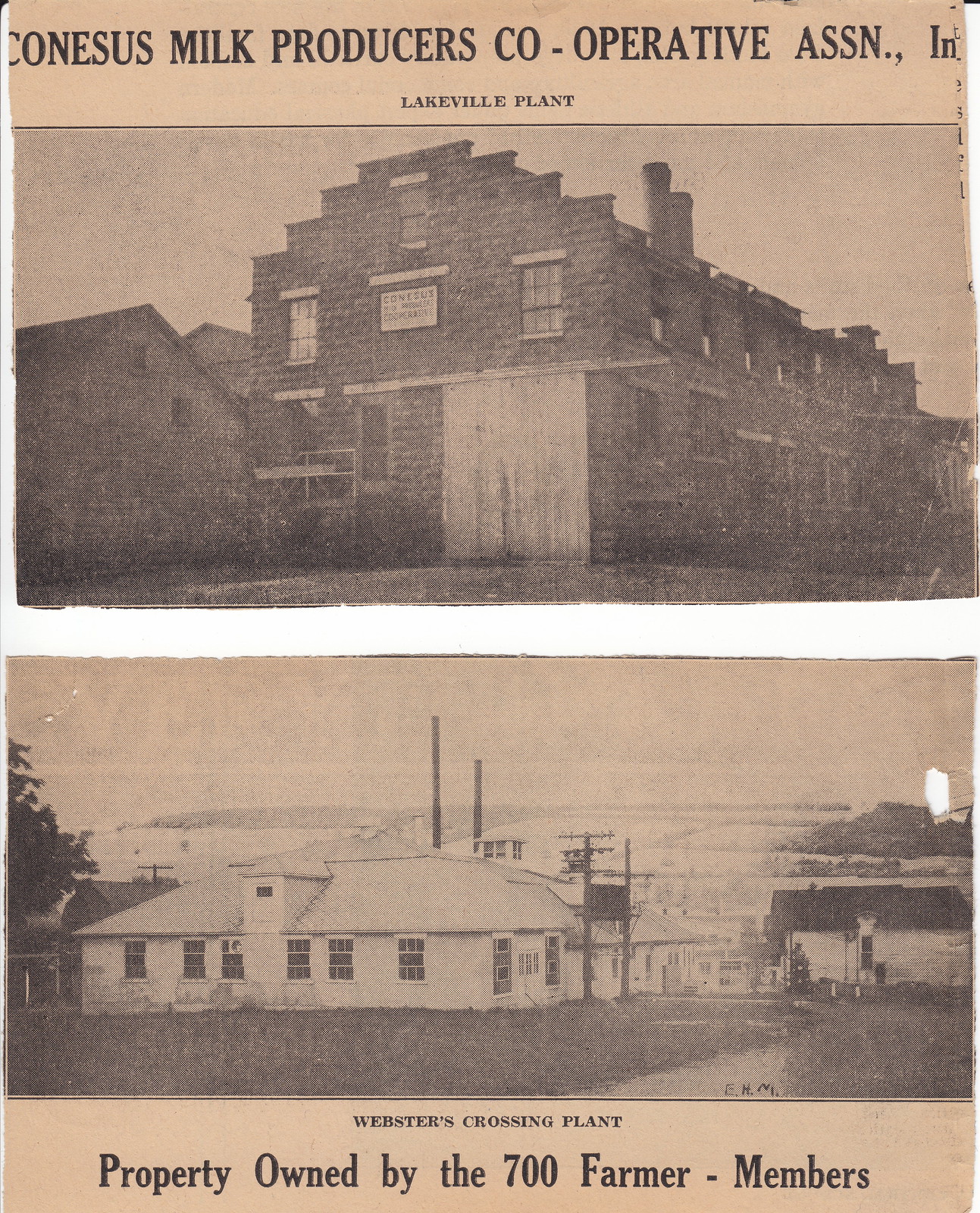The vintage image showcases an advertisement for the Canisius Milk Producers Cooperative Association. It features two sepia-toned photographs, each accompanied by descriptive text. At the top, a photograph of a large, multi-story brick building with a prominent white garage door and a chimney on the right is labeled “Canisius Milk Producers Cooperative Association, Inc. - Lakeville Plant.” To the left of this structure, a smaller brick building appears to be associated with the same company. Below this, a second photograph depicts the Webster's Crossing Plant, a smaller, white one-story building with a turret on the left. The surrounding area includes additional structures and what seems to be a body of water with an isthmus in the background. A tree can be seen on the left side of the image. The text beneath the second photograph proudly states that the property is owned by the 700 farmer-members. The photographs are separated by a white gap and have aged to a faded cream, indicating their historical nature.